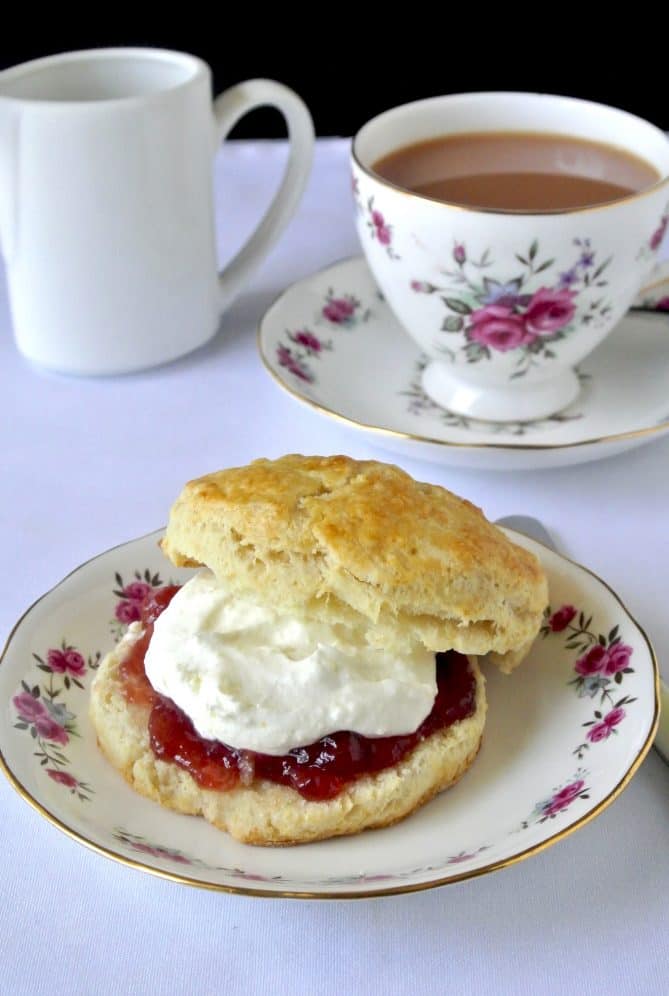The image depicts a beautifully arranged breakfast or tea-time setting. At the center, there is a small white circular plate with a gold trim and a floral design featuring pink flowers and green leaves around the edge. On the plate are two waffles, each topped with red jelly and a generous dollop of white cream, which might be cream cheese or mayonnaise. A bread and butter knife can be seen next to this plate. In the top right corner of the image, there is a cup of dark brown liquid, likely coffee or tea, placed on a matching saucer with the same floral design and gold trim. On the left side of the image, there's an additional white mug. The setup rests on a white tablecloth, and the overall brightness and clarity of the scene suggest a well-lit, inviting atmosphere conducive to enjoying a pleasant morning or afternoon meal.